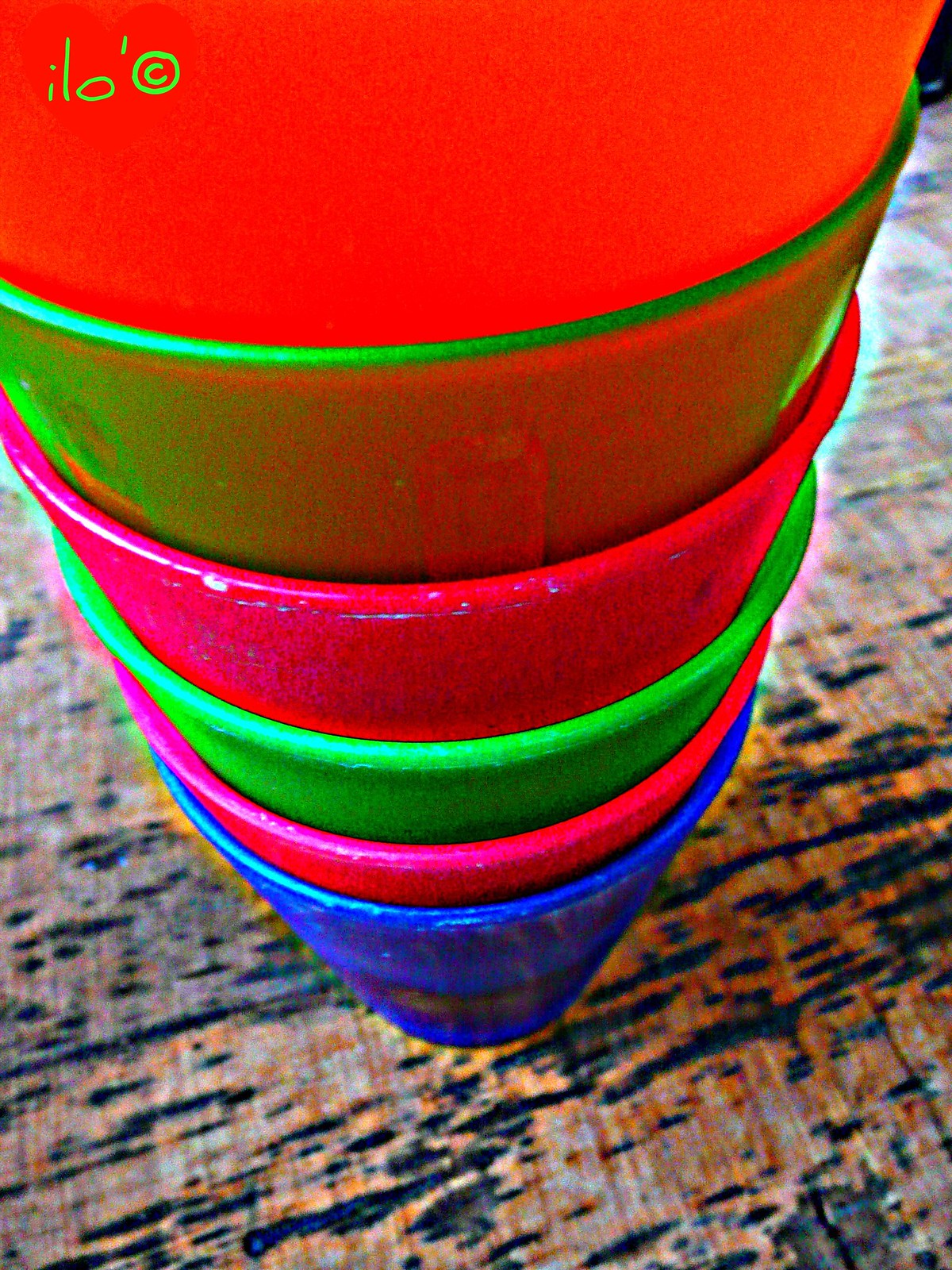This photograph captures a vibrant, oversaturated stack of colorful plastic cups or small bowls with a grainy, faded effect. The stack starts with a blue cup at the bottom, followed by a pink cup, a green cup, another pink cup, a second green cup, and finally, a red cup at the top, which almost encompasses the entire upper part of the image. The cups are stacked on a surface that seems to be a textile with a white base, crisscrossed sparsely by blue and yellow lines. In the top left corner of the photo, green text spells out "ILO" followed by an apostrophe and a copyright symbol enclosed in a circle.